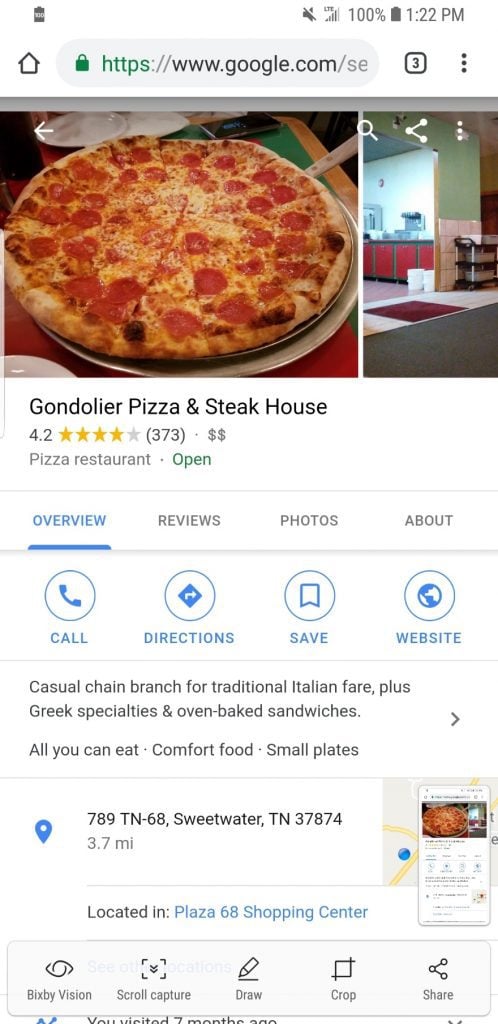A smartphone screen showing a search for restaurants. The top status bar displays the time as 1:22 PM, a full 100% battery, signal bars, and a "No Sound" icon on the upper-right side. Below that, the browser's address bar reads "google.com/..." which is partially obscured. The main content of the screen is a Google search result featuring an image of a pizza and an interior view of a restaurant labeled "Gondolier Pizza and Steakhouse." The restaurant has a 4.2-star rating based on 373 reviews and is categorized as a pizza restaurant with two dollar signs indicating moderate pricing. The restaurant is marked as open with a green indicator.

The result includes navigational tabs with "Overview" highlighted in blue, while "Reviews," "Photos," and "About" are in grey. Below these tabs, clickable blue icons for "Call," "Directions," "Save," and "Website" are available. A description of the restaurant follows, stating it is a casual chain branch serving traditional Italian fare, Greek specialties, oven-baked sandwiches, all-you-can-eat options, comfort foods, and small plates. 

Additional information includes the address "789 TN-68 Sweetwater, TN, 37874," located 3.7 miles away in the Pizza Plaza 68 Shopping Center. There is a vertical line dividing the content, with a small map view and smartphone interface on the right side of the screen.